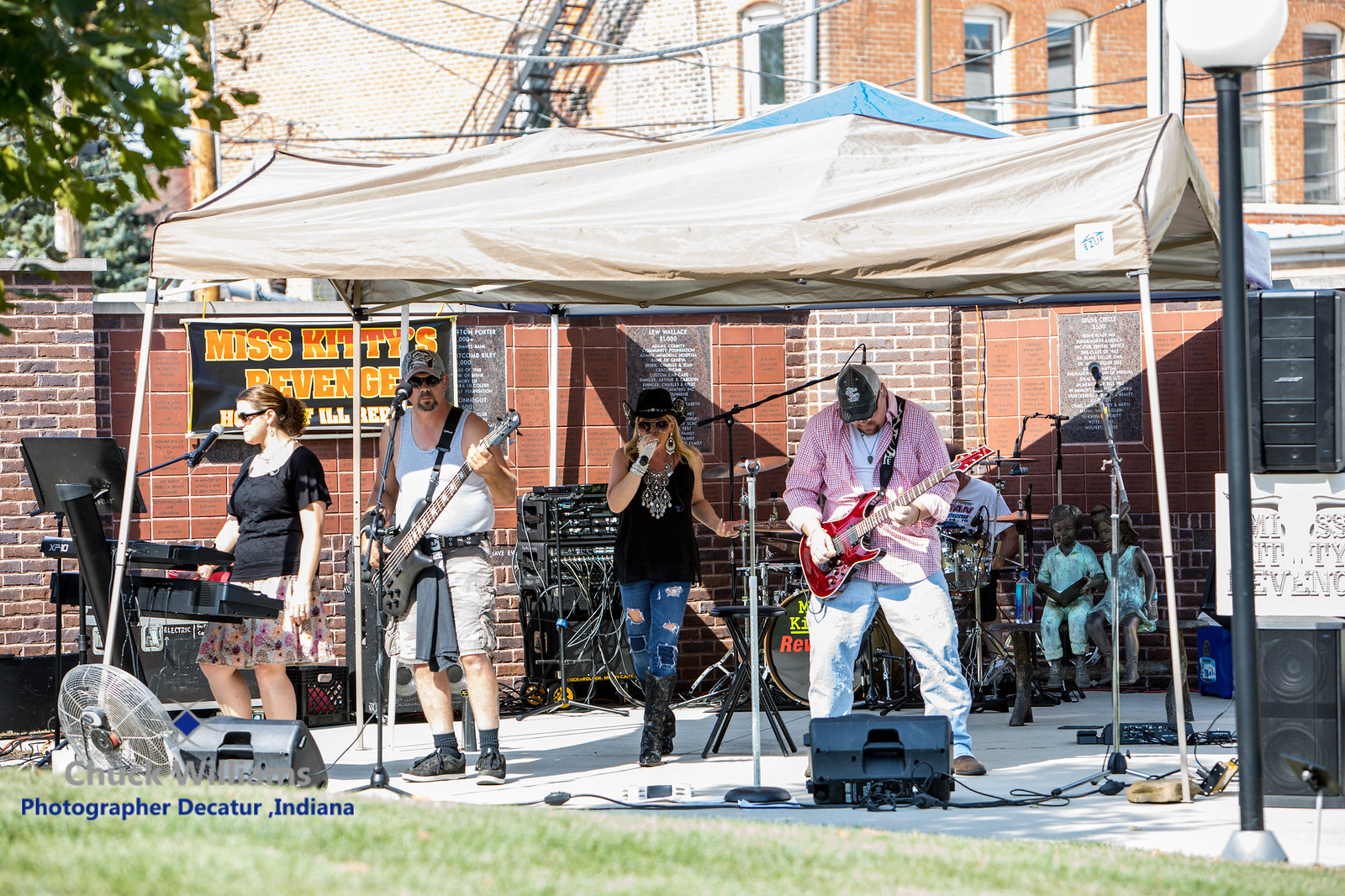A band is performing live in a downtown area on a bright, sunny day. The musicians are under a white pop-up tent set up on a concrete pad. On the far left stands a young woman with curly hair in a ponytail and a skirt, playing a keyboard and singing into a microphone on a stand. Beside her, a man dressed in a gray tank top, with a beer belly, is engrossed in playing an electric guitar. To his right, a young woman outfitted in a cowboy hat, ripped blue jeans, and tall boots holds a sparkly microphone, adding vocals to the performance. Another man, wearing a red and white button-up shirt with light blue jeans, is hunched over his red electric guitar, likely in the midst of a solo. In the background, partly obscured by the band and their sound equipment, there's a drum set and a man who appears to be playing it. Behind the drum set, statues of children seated on a bench add a unique backdrop to the scene. A photographer's credit at the bottom left corner reads "Chuck Williams, photographer, Decatur, Indiana."  The surrounding area features some green grass and additional sound equipment outside the tent, emphasizing the setting's casual, yet equipped nature.